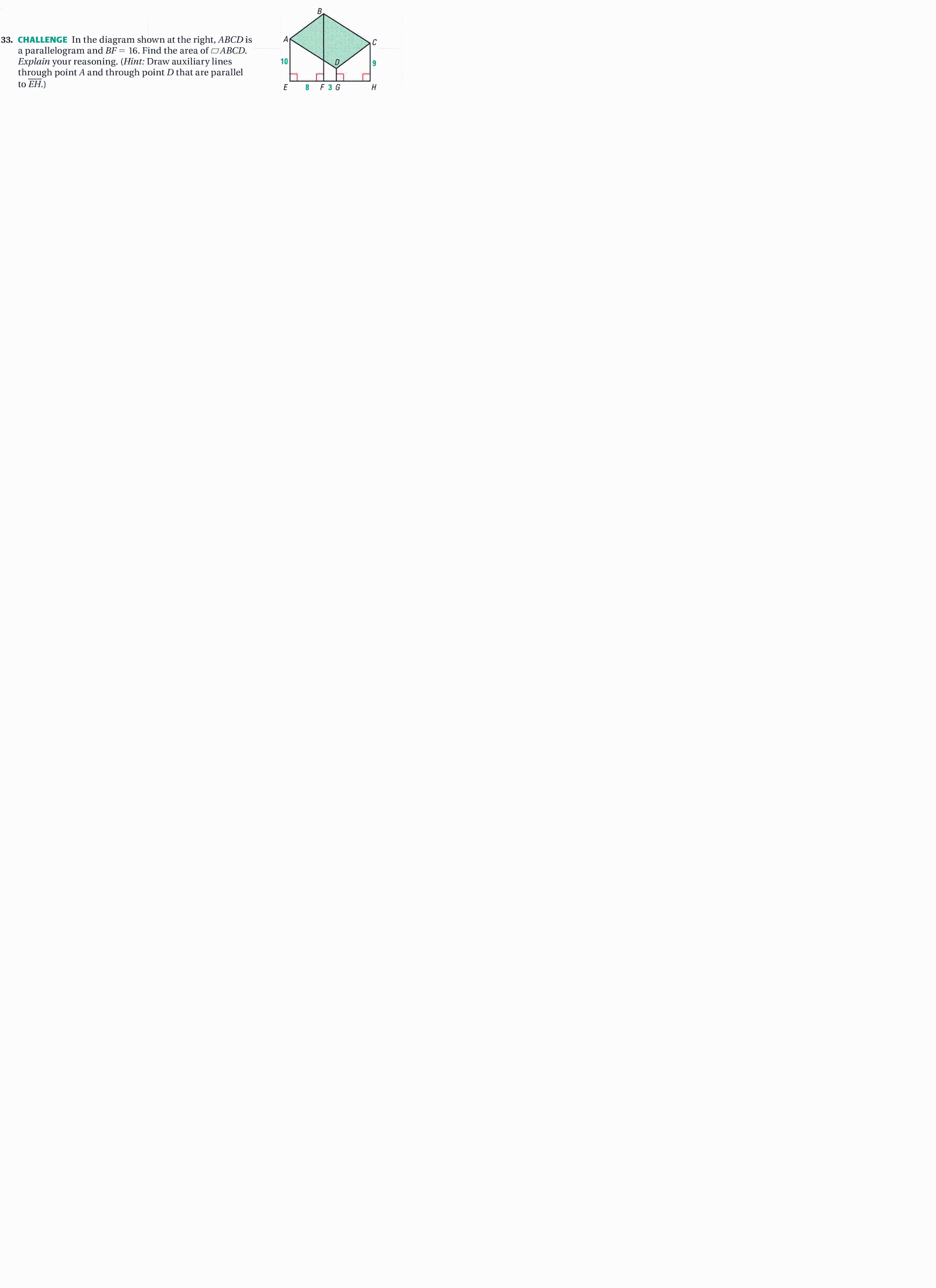A screenshot depicts a geometric problem involving a three-dimensional shape that appears to be part of a rectangular cube. Despite the tiny measurements that are difficult to discern, the image includes several dimensions marked along the edges of the shape. To the left of the cube, there is explanatory text, though it is too small and faint to be legible. The area of a rectangular section is highlighted in green, and some slight depth is indicated, suggesting a partially formed cube. The text and measurements are in black against a grayish background, making it hard to read at the current magnification.